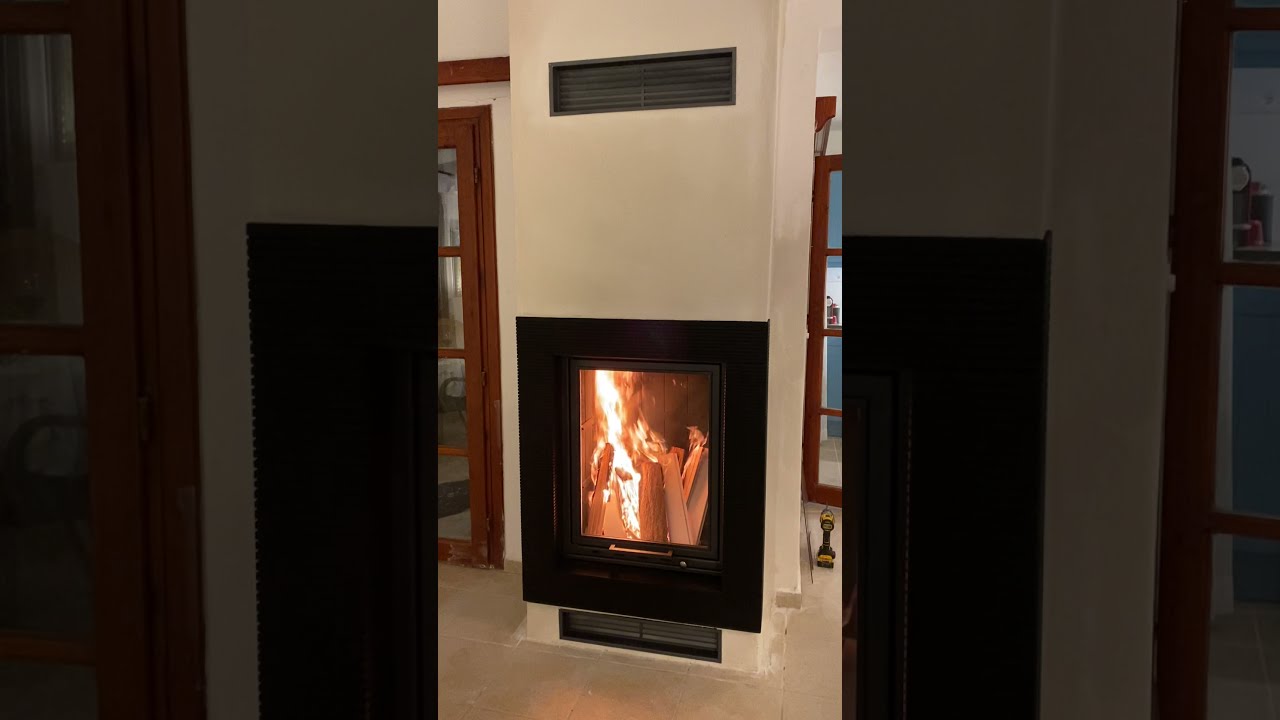In the center of the image is a black square fireplace filled with multiple cut logs that are actively burning, suggesting a warm, inviting atmosphere. The black fireplace is set into a white-painted wall, with a black vent located above it and another at the bottom, reinforcing its authentic functionality. The surrounding floor is adorned with various gray tiles, adding a modern touch. Flanking the fireplace are two doors, each framed in brown wood and featuring glass panels that create a mirrored effect. The white baseboards and door trims hint at ongoing construction or recent renovation. Notably, a yellow and black electric drill rests on the ground in the bottom right corner of the image, further emphasizing the work-in-progress state of the setting.